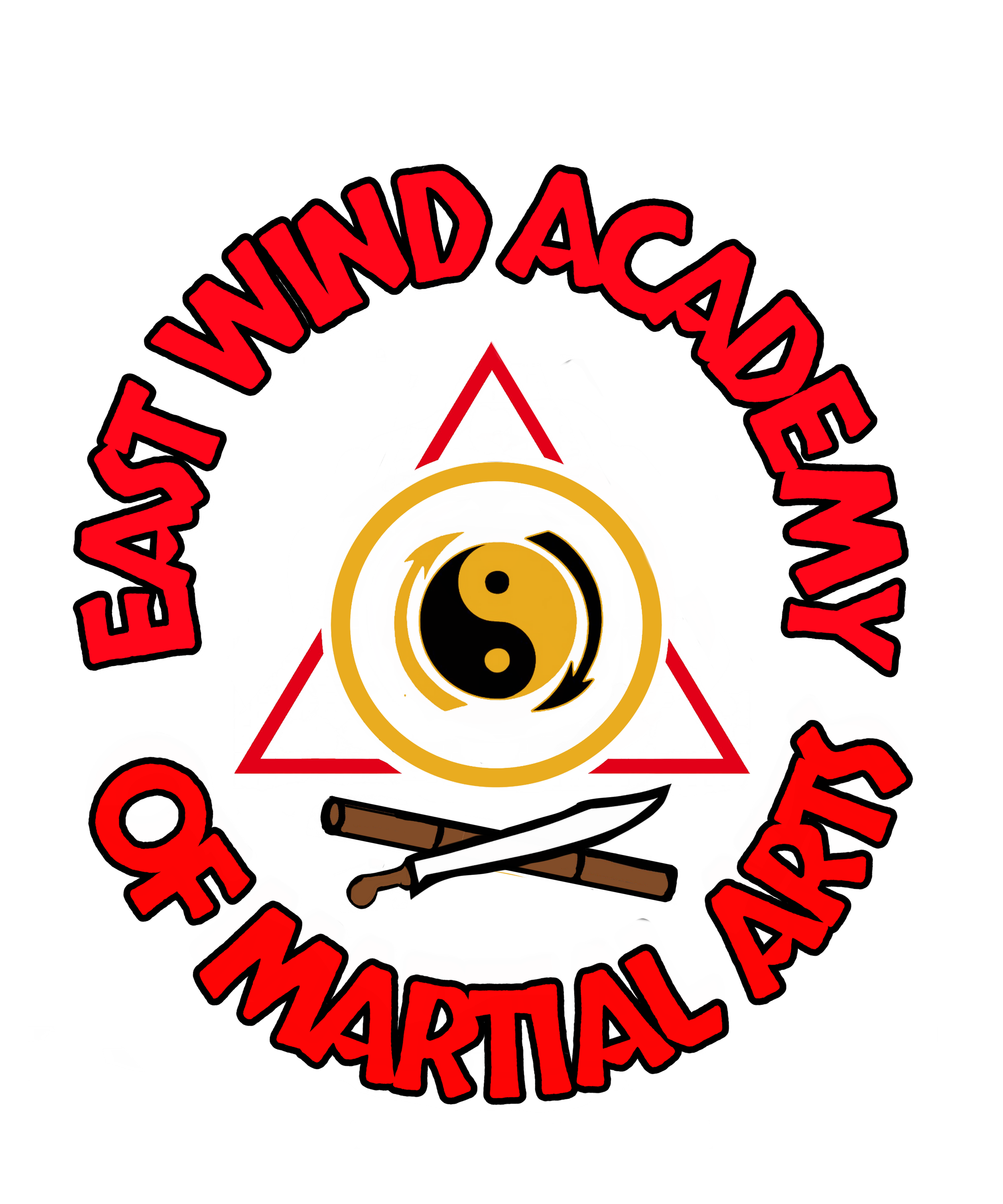The image is a detailed logo for "East Wind Academy of Martial Arts" presented without any background color or border. The text is bold, capitalized letters in red with black outlines, forming a circular or slightly oval shape around the logo. The words "East Wind Academy" arc along the top half while "Of Martial Arts" completes the bottom half.

At the center lies a complex logo: a red-bordered triangle houses a mustard-yellow circle. Nested inside this circle is a yin-yang symbol divided into mustard yellow and black sections. Two arrows encircle the yin-yang symbol, one pointing downward on the right and the other upward on the left, creating a clockwise motion. Below this central emblem, a sword and a wooden stick are crossed, adding further detail to the martial arts theme.